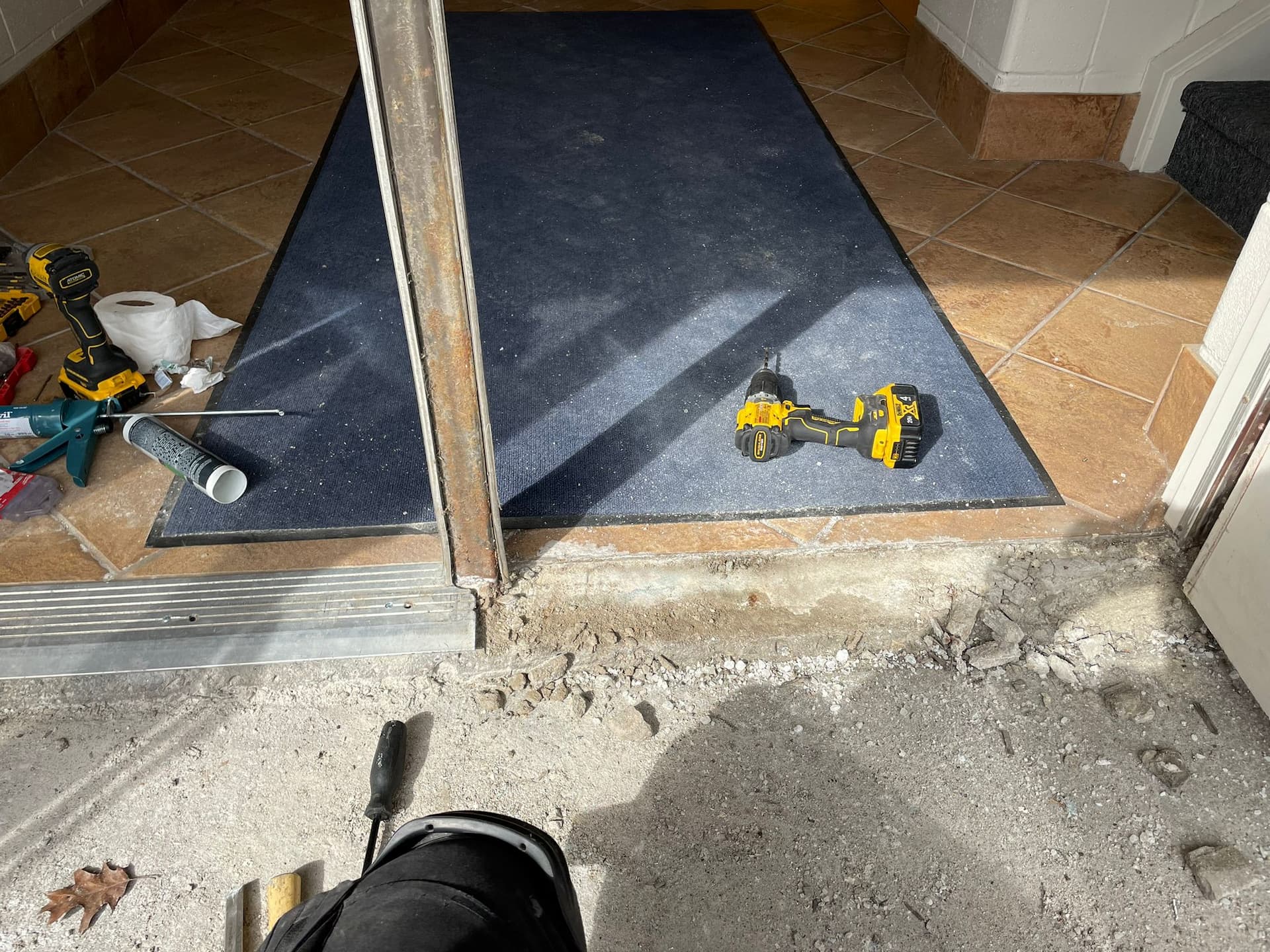In this photograph, we are outside looking in on a construction site of a new home. The foreground shows crumbling concrete, with a knee pad-clad knee and a black screwdriver lying on the ground. Ahead, a double door frame without the doors in place reveals the interior space. The door frame's metal threshold separates the exterior concrete from the interior beige tile floor. A long blue carpet runs into the room, partially visible under the threshold. On the right-hand side of the carpet, there is a yellow and black cordless drill. On the left-hand side, a collection of construction tools including another cordless drill, a green caulking gun, a white tube of caulk, and a roll of toilet paper is scattered about. Harsh sunlight casts shadows across the scene, highlighting the gritty, work-in-progress nature of the site.